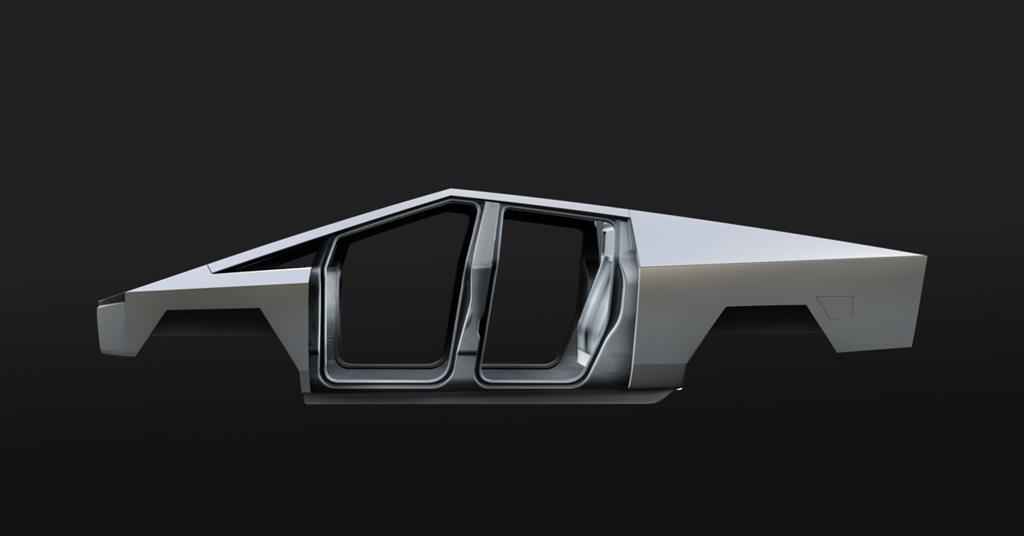The image showcases the sleek, unfinished stainless steel shell of a Tesla Cybertruck set against a stark black background, which makes the silver metal exterior pop. This contemporary, modern vehicle design highlights an angled, smooth roof, distinct cutouts where the tires, front, and back seats would be, and a visible gas compartment at the rear. The Cybertruck's outer frame lacks doors, wheels, a control panel, and interior seating, focusing the viewer's attention on its minimalist, futuristic outer design. The depiction is from a viewpoint facing the driver's side windows, emphasizing the clean lines and New Wave aesthetic of the vehicle's body.